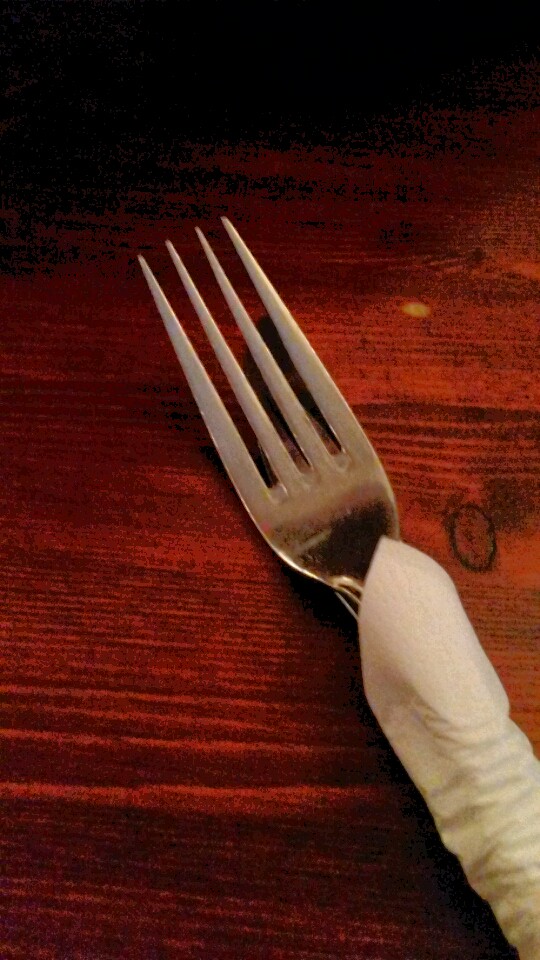This vertically cropped, grainy color photograph offers a close-up view of a fork partially wrapped in a white, slightly twisted napkin, coming in from the bottom right-hand corner with its tarnished tines pointing diagonally towards the upper left. The fork, which appears to have been used and is made of silver or stainless steel, possibly with some tarnish, is set against a dark honey-brown wooden table that showcases detailed grain patterns. The contrast between the metal of the fork and the wood's grain direction is stark, adding visual interest. The image, primarily in focus at the center, fades to darker tones towards the edges, emphasizing the fork and its surrounding textures. There's no printing or text within the image, contributing to its simplicity and focus on the mundane elegance of everyday tabletop settings.